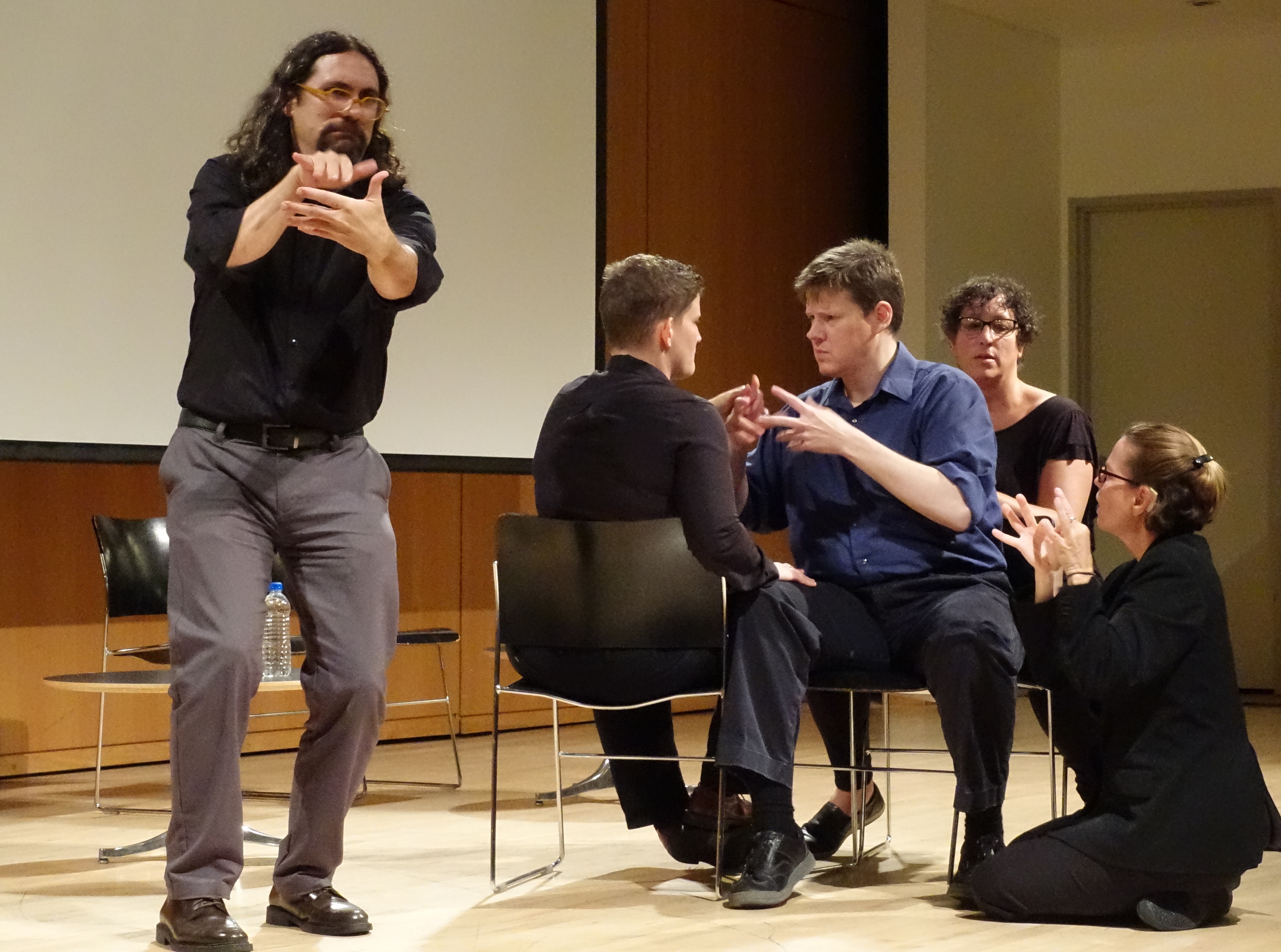In a classroom setting with beige and brown walls highlighted by wood paneling and a hardwood floor, a scene unfolds that appears to be an improv group or a sign language performance. Central to the scene is a man with long, curly brown hair, a goatee, and vivid yellow glasses. Dressed in a black button-up shirt, gray slacks, and black leather shoes, he stands in front of a large whiteboard and a projector screen, gesturing with his hands in a deliberate manner. Directly behind him are two empty plastic black chairs and a table holding a clear water bottle. 

To the right, four individuals are seated close together. Two men in buttoned-up shirts and dark pants face one another, engaged in hand gestures as they sit in black plastic chairs. Both have short brown hair, though one faces away while the other faces forward. Between them sits a woman on the ground with short curly hair, wire-rimmed glasses, and a black top, also engaging in hand movements. Further right, a woman with black-rimmed glasses, clad in a black coat and black pants, kneels on the floor, her hands raised and gesturing in unison with the group. Overhead lighting illuminates the scene, drawing attention to the intricacy of their hand movements against the backdrop of the classroom's projector and wood-paneled walls.